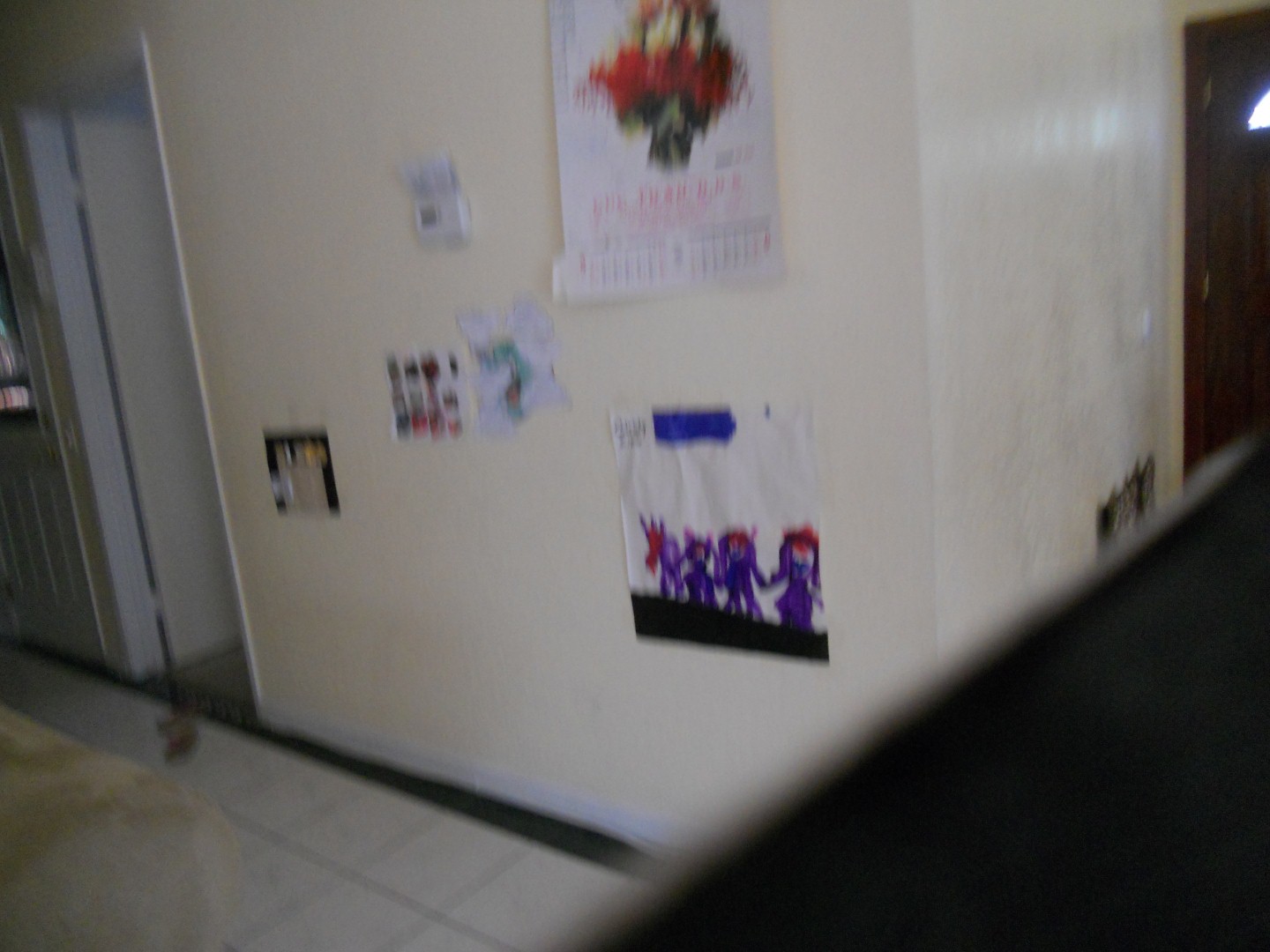This photograph, although blurry and inadvertent, captures an interior corner of a house or apartment hallway. The white walls, adorned with childlike drawings and posters, give a sense of a family-friendly environment. Specifically, there are drawings of purple figures with red hair, a flower basket, and other indistinguishable artwork. A white tile or linoleum floor continues the light, neutral color scheme, complemented by white trim. Notable on the wall is a white thermostat or air-conditioning controller, along with what seems to be a calendar positioned higher up. The open white door leads to another part of the hallway, which curves to the left where a brown door can be spotted, potentially the entrance to another room. A gray ledge is present in the foreground, adding depth to the image. Despite its blurriness, the photograph provides a snapshot of a cozy, child-friendly home with practical and personal touches.